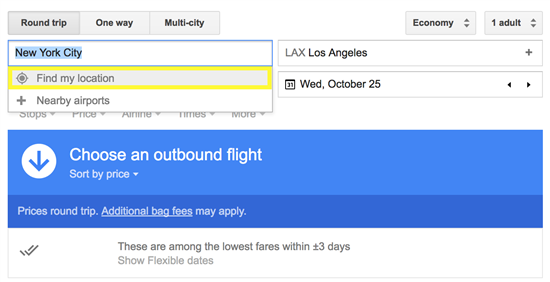The image is a partial screenshot from a travel website, capturing the top one-third of the page. Here's a detailed view of the elements visible:

- **Menu Bar**: At the very top, a navigation menu is displayed, but no company name is visible. The menu options suggest it’s a flight booking site, offering choices like "Round-trip," "One-way," and "Multi-city" displayed from left to right. On the far right, there are settings for "Economy" class and "One adult" passenger.

- **Flight Search Fields**: The primary section for entering flight details shows that the user is searching for flights. There are text boxes indicating:
  - **Departure City**: "New York City" is entered in the departure field, which is highlighted in blue. Below this field, a yellow rectangle outlines the option "Find my location." Additionally, there is a "+" sign next to "Nearby airports."
  - **Destination City**: "LAX, Los Angeles" is entered as the destination.

- **Date Selection**: Below the destination field, the date "Wednesday, October 25th" is displayed within a white-background rectangle.

- **Flight Selection Section**: The section for choosing flights has several elements:
  - A blue bar with a white circle containing a blue downward arrow. The text in white reads "Choose an outbound flight."
  - Below this, there is an option to "Sort by price," indicated by an inverted white triangle, suggesting a drop-down menu.
  - The phrase "Price is round trip" is written in a slightly darker blue rectangle, underlined, with a white note stating "additional bag fees may apply."

The overall background of the page is white, enhancing the visibility of the highlighted sections in blue and the text presented.